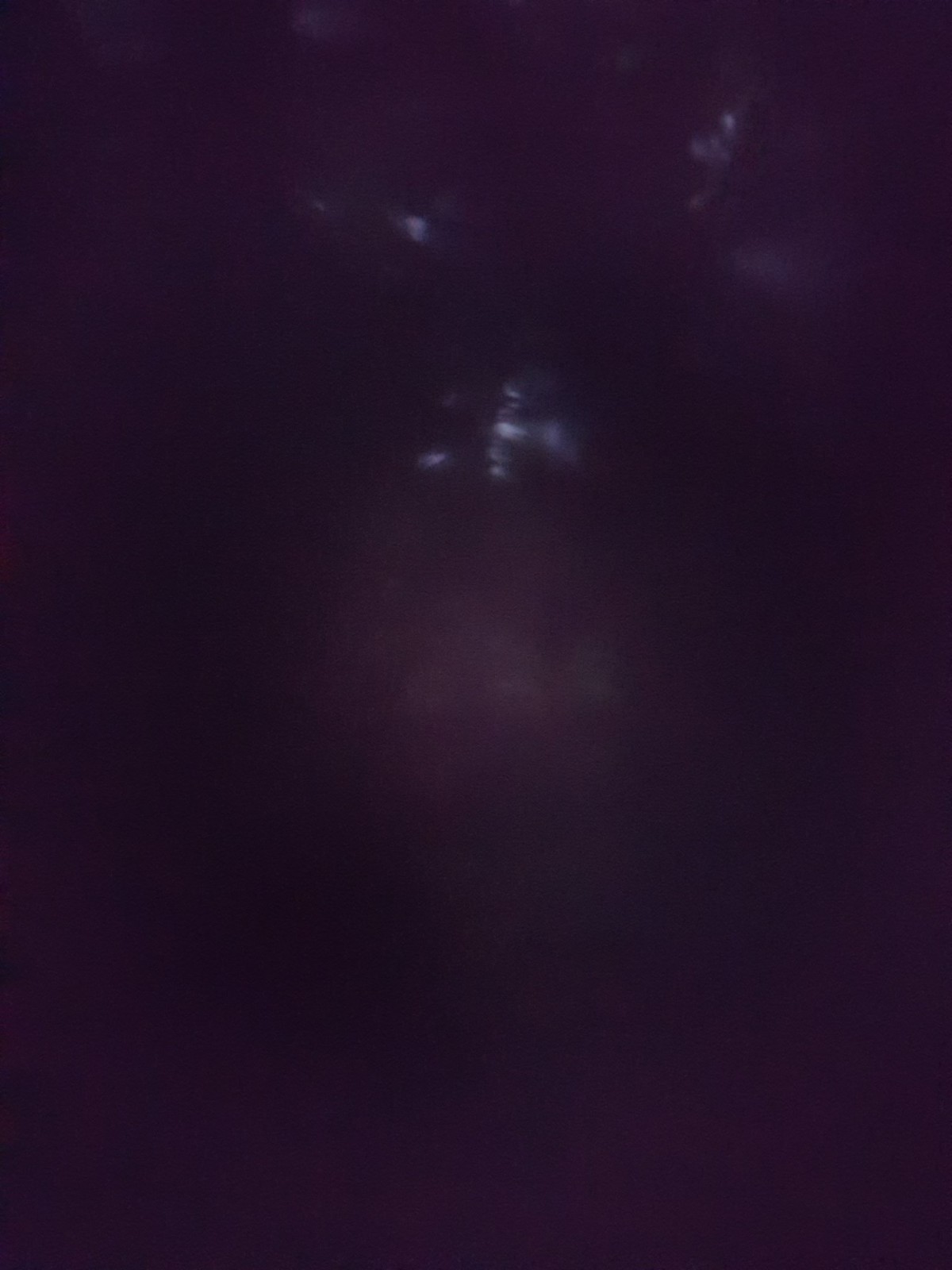This photograph appears to have been taken at night in a setting with minimal to no lighting, rendering most of the image completely dark. The majority of the picture is enveloped in blackness, making it almost impossible to discern the subject matter. However, towards the center and stretching towards the top, there are faint and scattered reflections of light. These reflections might be glinting off a surface like a plastic bag or something similar, but the vague illumination makes it challenging to determine the exact nature of the object captured. The light reflections could also suggest water or another reflective surface, although the lack of clarity leaves the true subject of the photograph ambiguous.